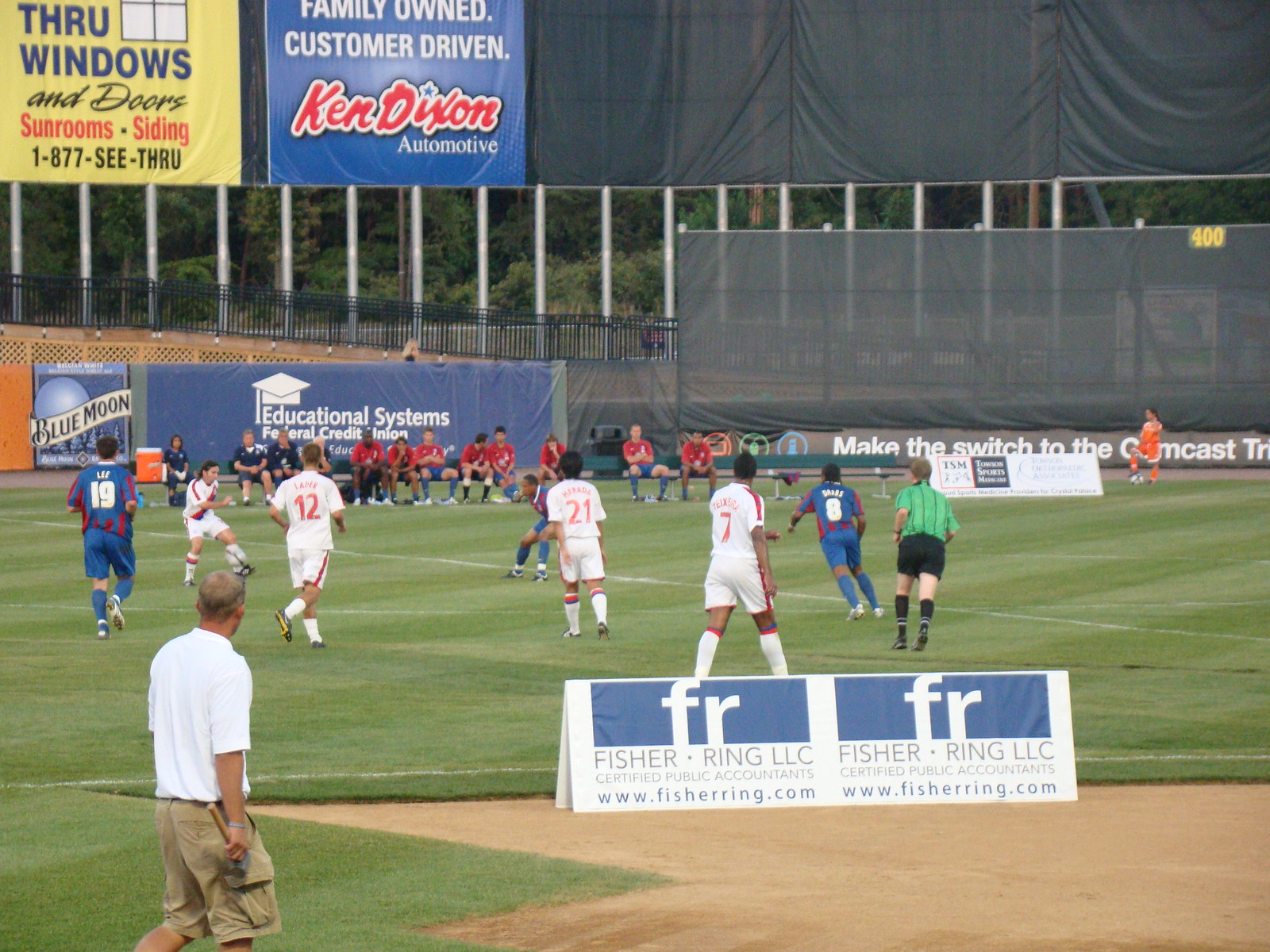The image captures a vibrant soccer match in an arena adorned with various banners and advertisements. The field, meticulously striped with white paint, is surrounded by green grass and dotted with signs, including one from "FR Fisher Ring, LLC" featuring a blue background with white lettering. The scene features two teams: one in white uniforms with red accents, and the other in blue uniforms with red accents, both competing intensely. Along the grandstand, banners add to the lively atmosphere, such as a prominent yellow banner and a bold blue banner. Additional advertisements around the arena include promotions for educational systems, Ken Dixon Automotive, and Saunders and Seiding. On the sidelines, a team in red short-sleeved jerseys and blue shorts sits on benches, while a referee in black shorts and a green shirt oversees the game. Among the onlookers, a man in a white shirt and beige shorts walks just outside the field’s border. To top it off, a large banner promoting Comcast reads, "Make the Switch to Comcast," standing out in the background of this dynamic scene.